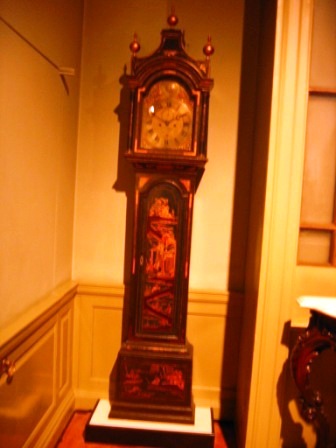This color photograph features a grandiose grandfather clock positioned centrally, dominating the scene from bottom to top. The clock is slightly out of focus, adding a nostalgic ambience. The wooden case has a rich reddish hue, possibly highlighted by the lighting in the room. The top of the clock showcases a distinct design with three ornate tips crowning its apex.

Within the clock’s upper section, intricate metal components are visible, indicating the clock's face and operational elements. Moving downward, the clock’s transparent lower portion reveals its mechanical innards, offering a glimpse into the precision engineering within. The clock’s base is broader, providing stability and grandeur.

The entire clock sits on a platform with a contrasting white top and black border, nestled into a recessed nook in the wall. The surrounding walls are painted an inviting orangey hue, further complemented by a wooden baseboard that runs along the bottom, adding warmth and a homely touch to the setting.